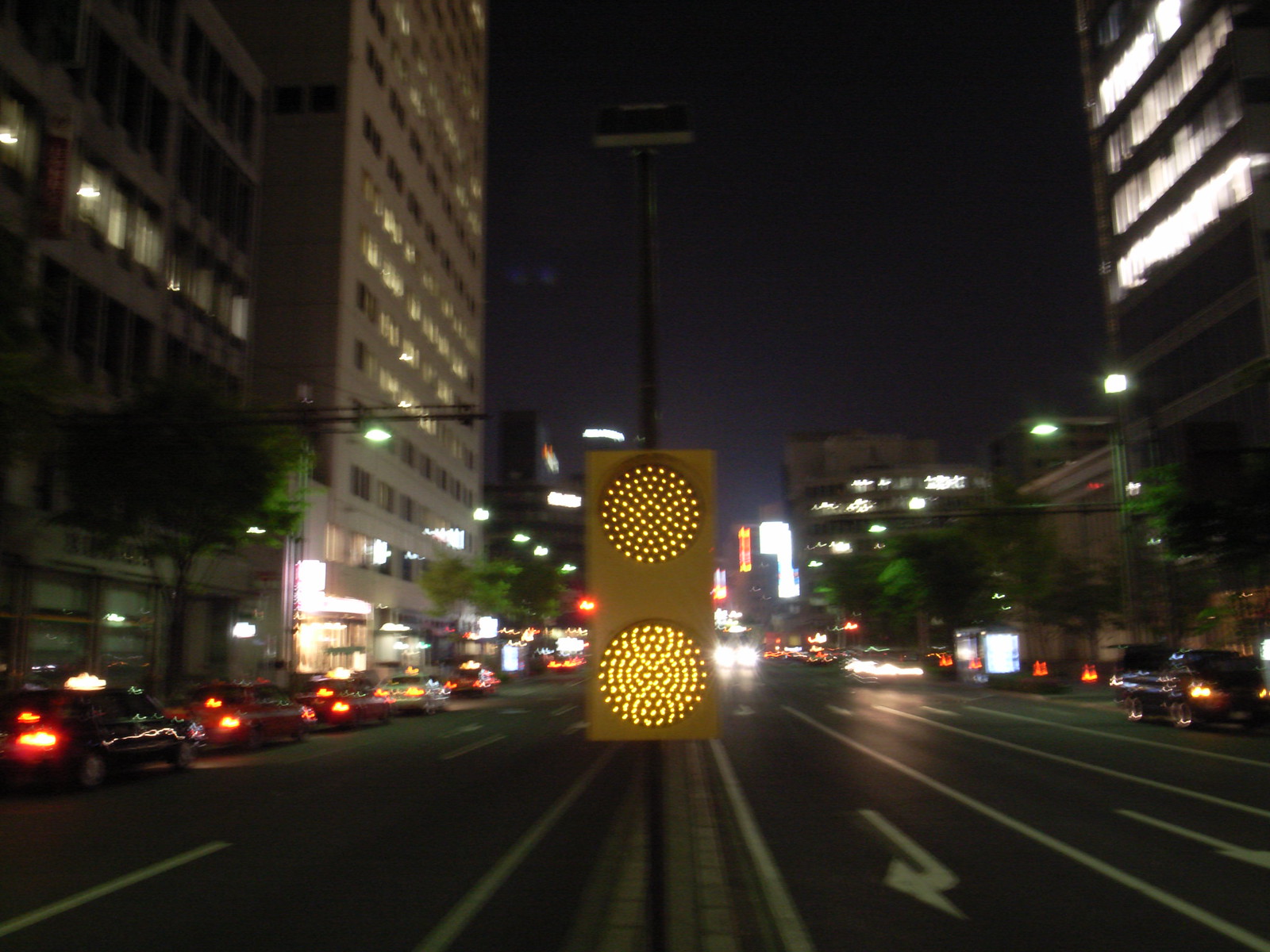A nighttime photograph captures a city street scene. The pavement is a muted gray, intersected by crisp white lane markers. The perspective of the image reveals oncoming traffic, indicated by directional arrows painted on the road. In the distance, a car approaches with its headlights brightly illuminating the way, while another vehicle seems to be on a similar path, drawing nearer. Off to the right, a car is visible with only its running lights on, adding a subtle glow to the scene. Dominating the center of the image is a gold-colored, rectangular stoplight with two glowing lights. This stoplight, positioned on a median that separates the street, stands as the focal point, its purpose unclear but its presence undeniable.